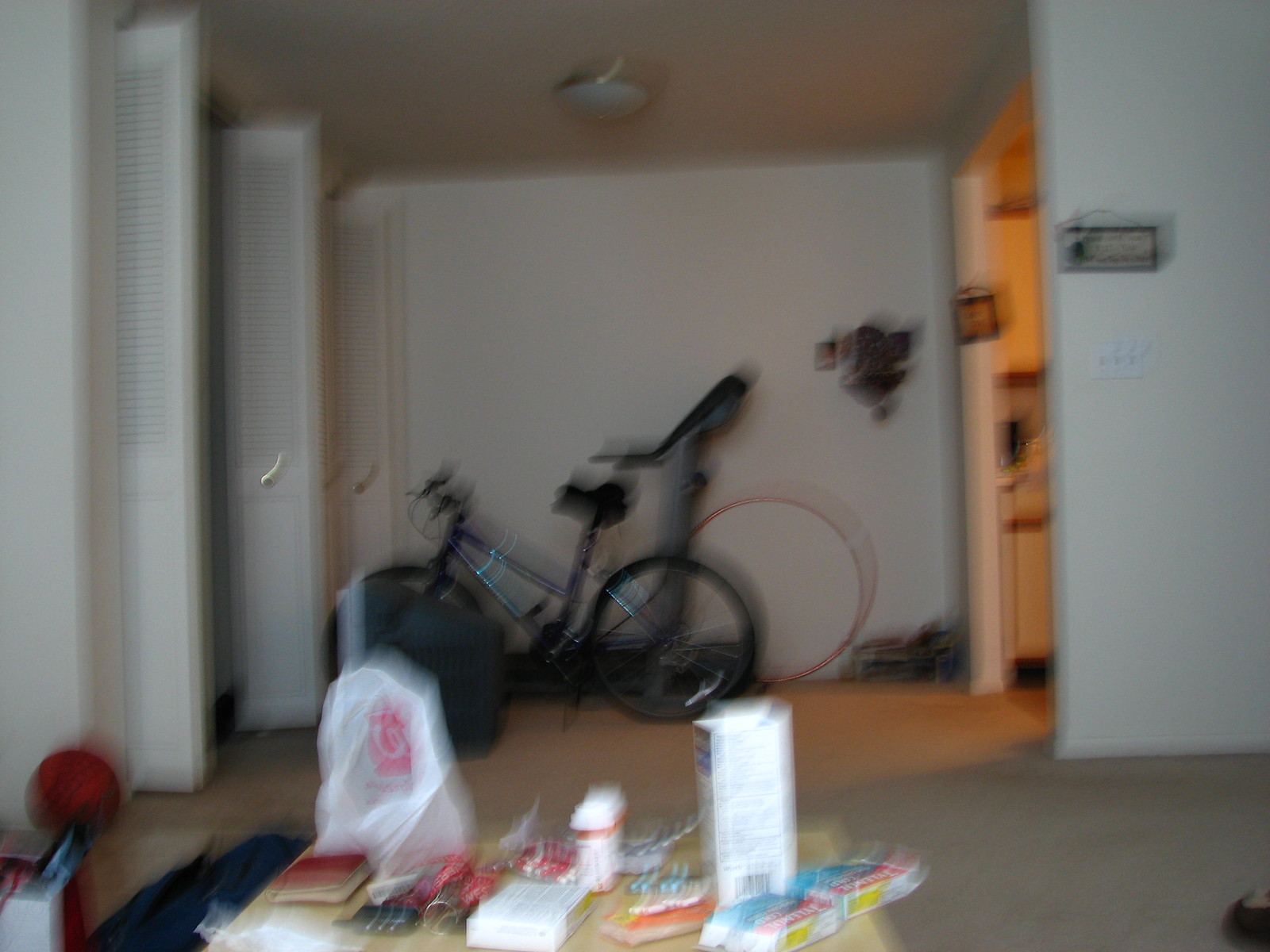This close-up photograph displays a living room setting with detailed observations, though the image is blurry. The foreground features a light brown coffee table cluttered with various items: a clear bag branded with the Walgreens logo, a maroon book, orange cylindrical pill bottles with white lids, and some paper pieces along with other boxes. One notable box is cyan and red with a yellow tag on the back. Scattered on the table are keys with an alarm fob, an orange and red push-out foil, and a white bag with red font. The room's walls are white, and the carpet is a cream-colored tan. 

In the background, there is a black bicycle leaning against a gray treadmill. Both the bicycle and treadmill partially obscure each other. The black treadmill has silver spokes visible on its front. A white wall with something dark hanging on it serves as the backdrop. To the left, there are closet doors with ventilation holes and gold-colored lever handles. The right side of the room opens to an illuminated kitchen, with light coming from fluorescent lighting, providing a golden hue to the secondary space. In the left corner, a red ball is faintly visible, adding a minor splash of color to the scene. Despite the image's blurriness, it captures a domestic space transitioning into a kitchen area with considerable detail.